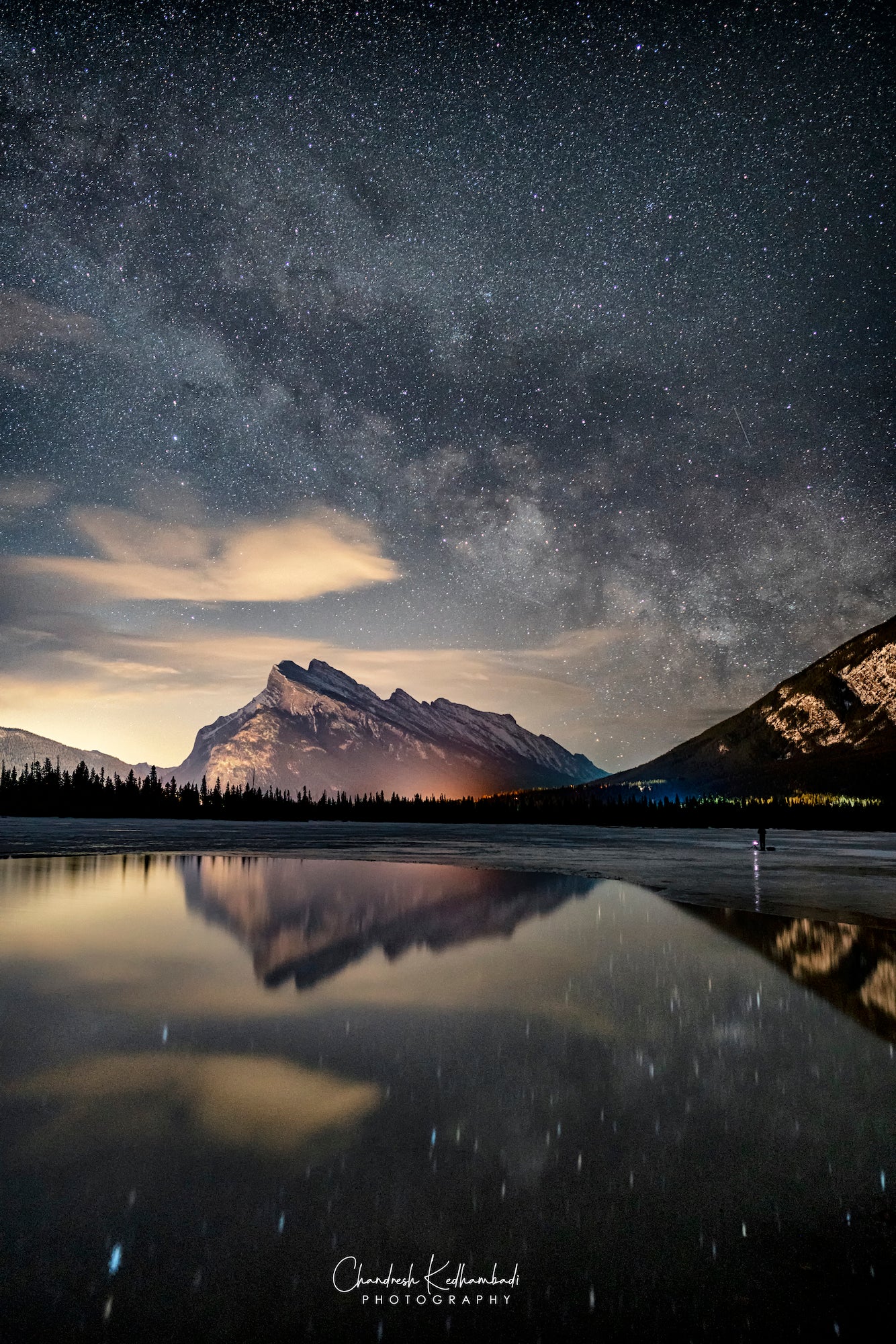A breathtaking nighttime landscape photograph captures the majestic Milky Way in all its glory. The sky, dark blue and filled with thousands of stars and a couple of distant clouds, spans two-thirds of the image, creating a dense canopy of constellations. A slight golden hue from a residual sunset tints the horizon, adding a delicate splash of color. Below, a pristine lake mirrors the celestial spectacle above, with its serene, glass-like surface transitioning to choppier, grayish-blue waters further afield. The opposite shoreline features a dense line of tall pine trees, all backlit and silhouetted against the starry sky. Centered in the image is a formidable mountain, its jagged peaks adorned with patches of white snow and green foliage, embodying the rugged beauty of nature. To the right, another mountain with dense greens and exposed gray rock slopes downward. The reflection in the water creates a seamless continuation of the landscape, making the scene even more mesmerizing. An inscription at the bottom in cursive, with the word 'photography' clearly visible, credits the photographer for capturing this awe-inspiring natural panorama.